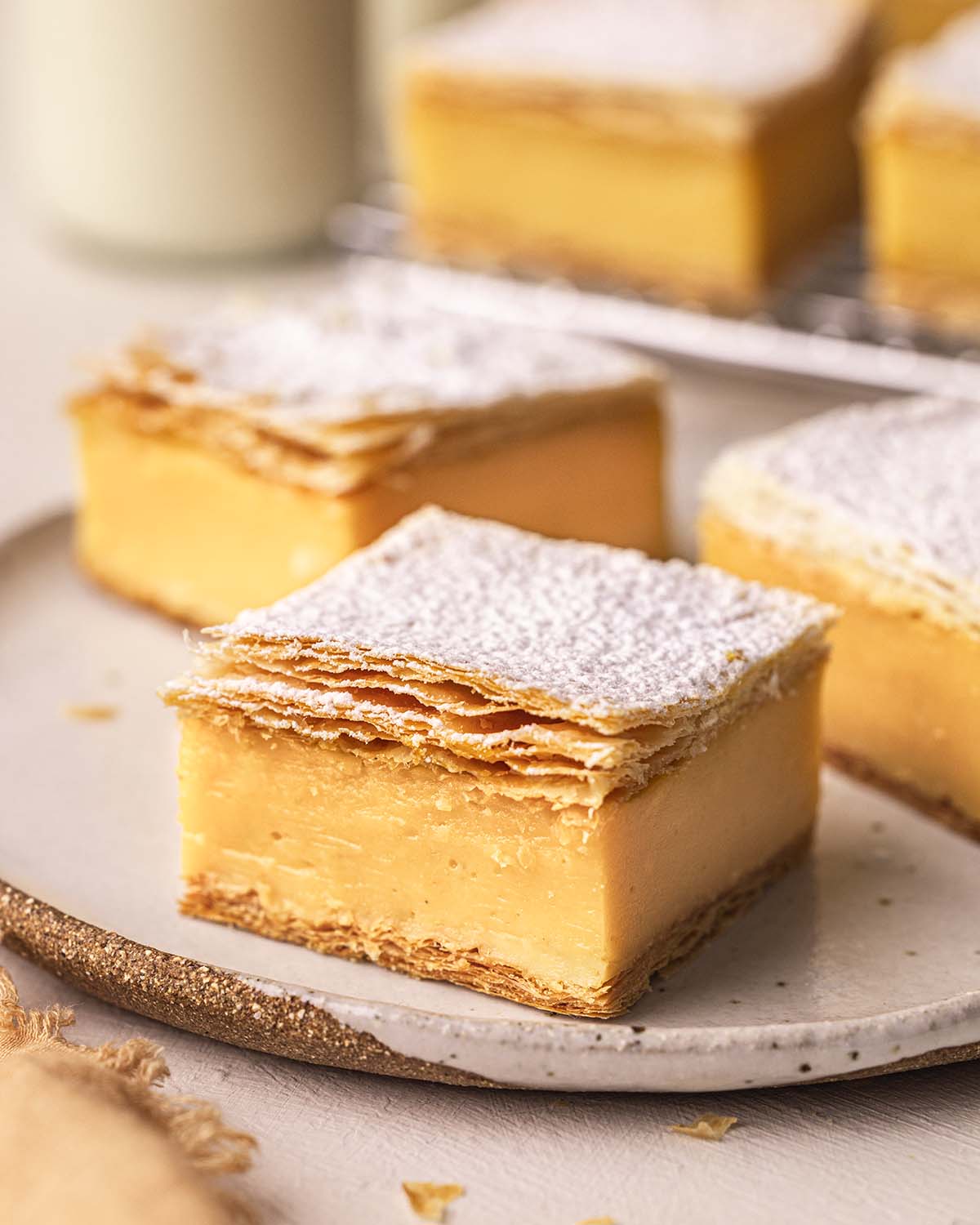The image showcases a beautifully arranged tray of square-shaped dessert items, resembling cakes or pastries. These delectable treats appear to be butterscotch or caramel brownies, each consisting of a flaky pastry base, a thick layer of orangish or light brown cream filling, and a flaky top dusted with powdered sugar. They are all meticulously positioned on a circular white plate, which rests on a white table. The central portion of the image features three prominently displayed pieces in the foreground, with additional blurred slices visible in the background, enhancing the overall presentation. The color palette of the image includes butterscotch brown, white, gray, and black, contributing to the delicious and inviting appearance of the sweet treats.